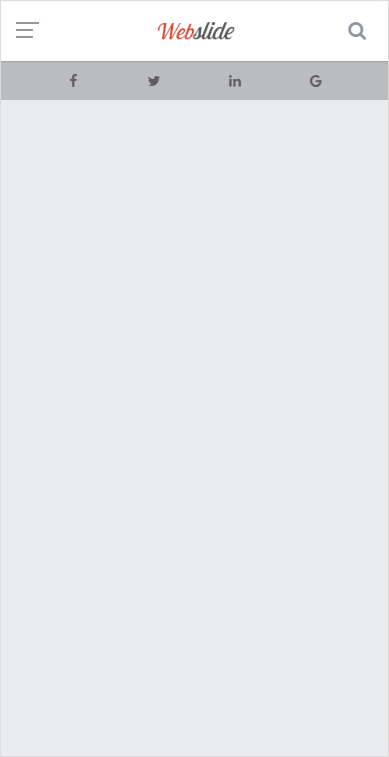In this image, we observe a detailed design layout with various graphical elements. 

At the top, there's a grey outlined block set against a white background. Towards the far left of this block, we see three horizontal grey lines, with the topmost line being the longest, and the bottom two lines significantly shorter.

Centered within the block, the text "Web Slide" is prominently displayed. The word "Web" is written in bold red letters, while "Slide" is in bold black letters. Adjacent to this text, on the far right, is a grey magnifying glass icon symbolizing a search function. 

Beneath this line of text, there's another block outlined in grey. Spanning from left to right are a series of black font logos. The first logo is Facebook's recognizable "F." Following that is the Twitter logo, represented by a bird now dubbed "Hex the Bird." The third logo, featuring the letters "IN," denotes Indeed. Finally, the fourth logo, a stylized "G," signifies Google.

The subsequent block below this array of logos consists of a light grey square. This section is devoid of any text or images, presenting an unobstructed light grey background.